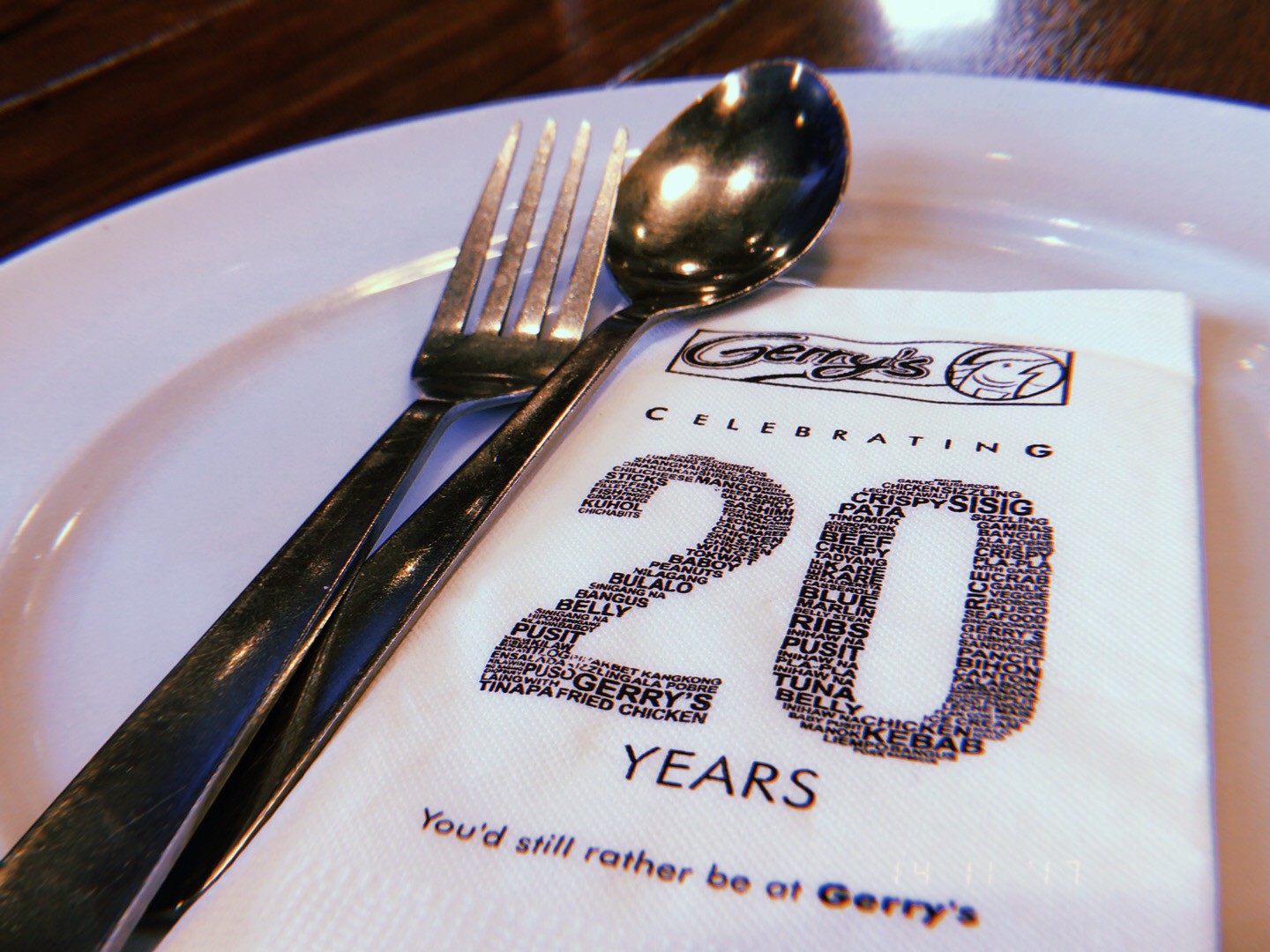The photograph, taken indoors, features a close-up view of a white China plate situated on a dark brown walnut table. The table is visible starting at the upper left-hand corner, extending down about an inch on the left and about half an inch on the right side. The curved top of the plate is in view, while its left, bottom, and right edges extend off-screen. Centered on the plate at a rightward angle is a white napkin. At the top of the napkin is a black-outlined rectangle with the name "Jerry's" accompanied by a logo of a marlin fish head. Beneath this, the napkin reads, "Celebrating 20 years" in large numbers, with the "2" and "0" cleverly designed using a list of menu items such as chicken, ribs, and kebab. The tagline "you'd still rather be at Jerry's" is printed at the bottom. To the left of the napkin sits a silver spoon, and next to the spoon is a matching silver fork.